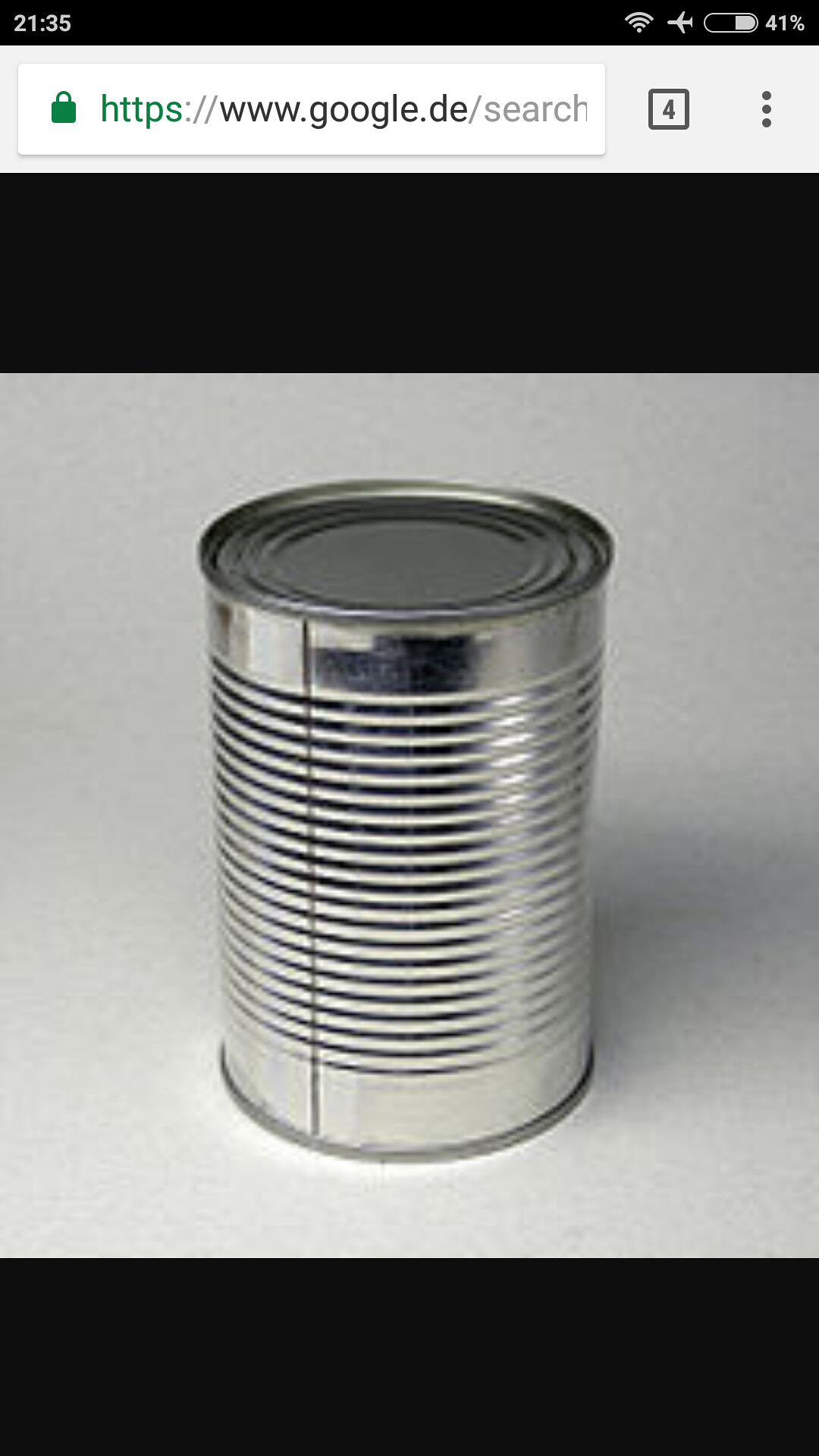This image showcases a silver can placed on a whitish-gray surface. The can is sleek and smooth at the top while the body features evenly spaced, ribbed circles running horizontally around it. A distinct black vertical line runs from the top to the bottom on the left side of the can. The photo appears to be a screenshot taken on a smartphone, as evidenced by the Google search bar visible at the top, displaying the URL "https://www.google.de/search" and a "4" in a small box next to it. Additionally, three vertical dots are visible, indicating more options. The image is framed with black strips at the top and bottom, possibly added to enhance the composition.